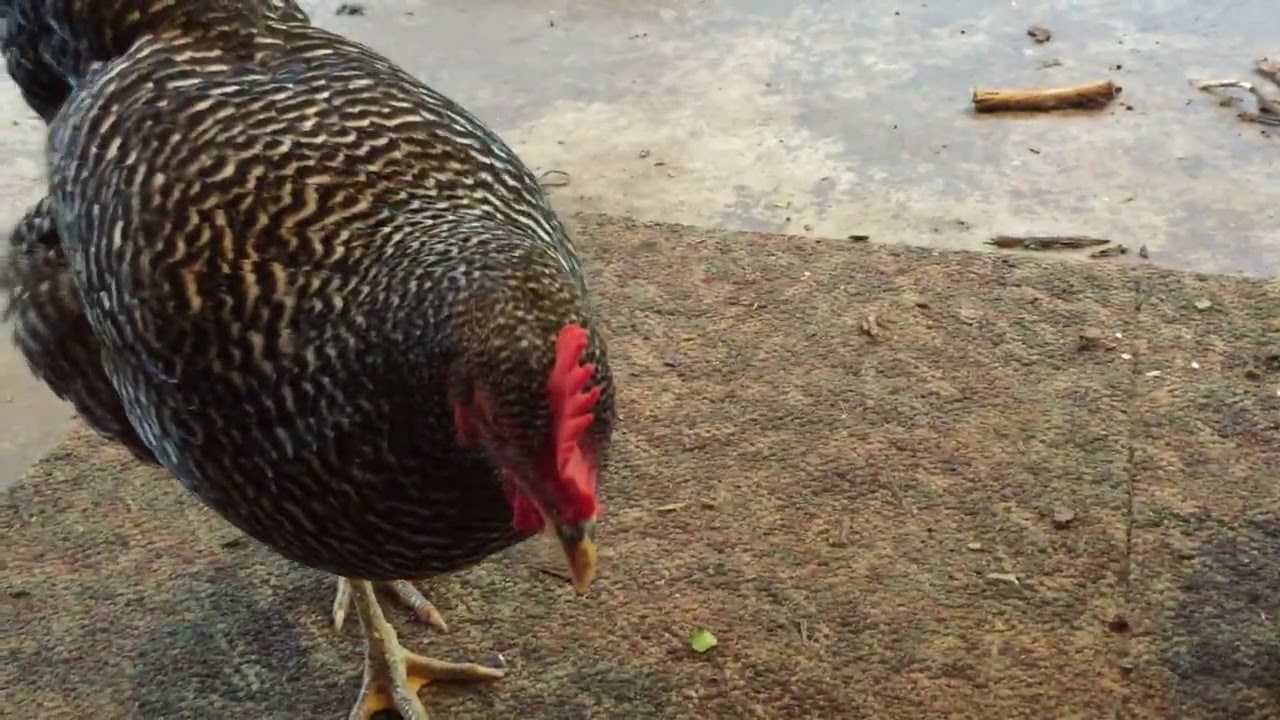The photograph features a prominent, vibrant rooster set against a rustic background. The rooster, showcasing its bright red comb and wattles, stands on a dirty, brown carpet that mimics the color and texture of soil, extending over a cement floor with scattered debris and rocks. The rooster’s plumage is a striking marbled pattern of black and white, with its head directed downward as if foraging for food, possibly seeds or small nuts. The scene also includes hints of greenery, such as a small piece of a green leaf nearby. Dominating the left side of the image, the rooster's yellow beak and feet are visible, although the bird seems more engaged in its search than in the presence of the camera. The background extends into a cement area with blotchy patches and scattered items like sticks and stones, giving the entire setting a raw, unkempt appearance.